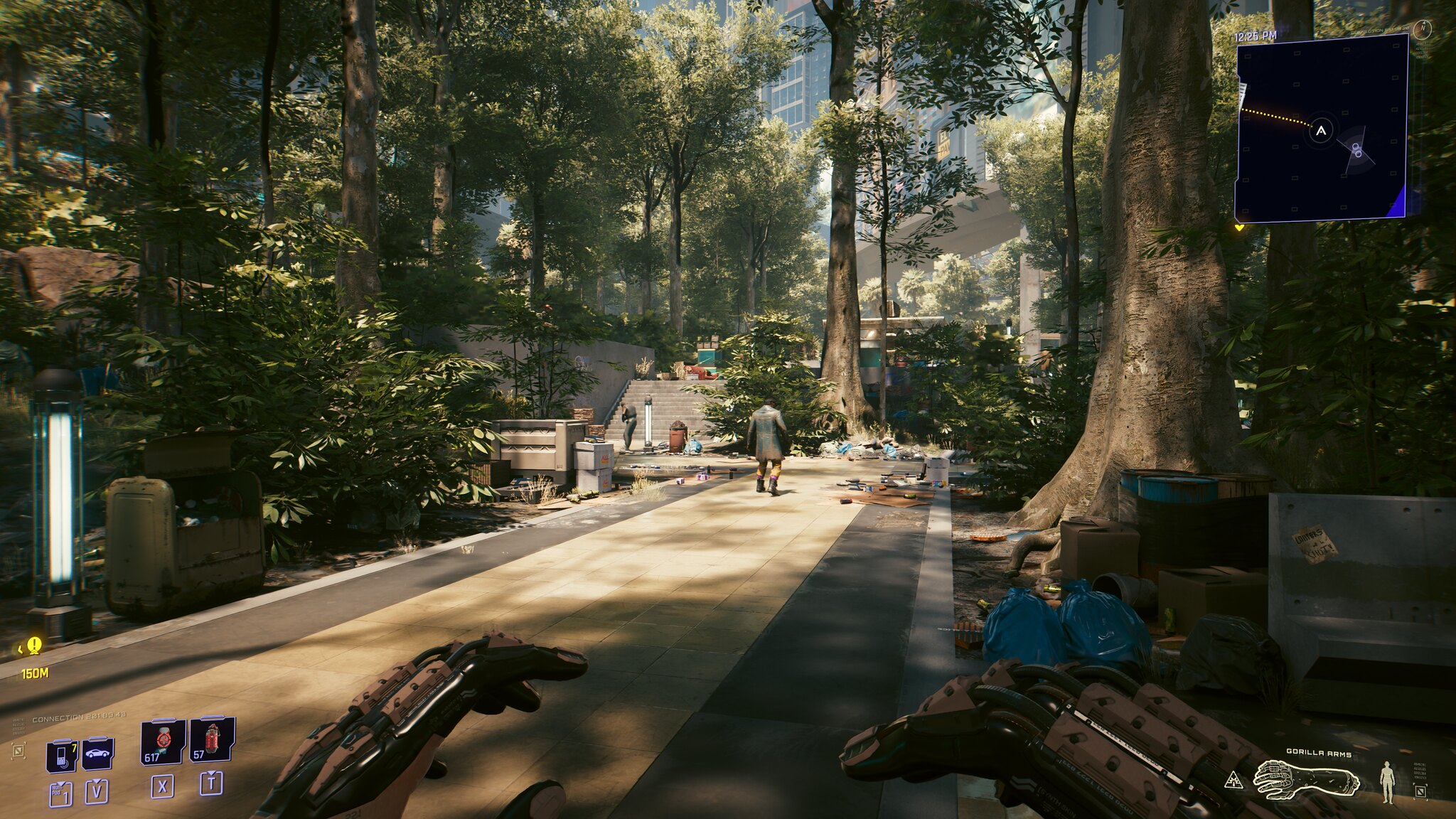A screenshot from a modern, high-definition video game captures an immersive forest scene. In the foreground, a tan path emerges from the lower left corner, winding back and then taking a sharp 90-degree turn to the left, leading out of sight into the dense background. Along this path, a solitary figure is visible, walking away toward the horizon. Dominating the scene are massive tree trunks—one prominently in the center background marks the end of the path, while another, towering and closer to the foreground on the right, stretches upwards beyond the frame. 

The left side of the image is thick with trees, creating a dense woodland atmosphere. In stark contrast, a distant city skyline with towering skyscrapers peeks through the central background, juxtaposing nature with urban elements. Closer to the foreground, scattered buildings hint at a transitional zone between the forest and the city.

Adding to the game's intricate design, mechanical appendages, resembling large brown hands, extend from the left and right near the center of the screen, suggesting a blend of organic and technological elements. Small video game overlay icons are neatly arranged in tiny square boxes on both the left and right sides of the screen, maintaining a minimalist interface. Notably, the image is absent of any words, text, or other descriptive text, allowing the visual elements to speak for themselves.